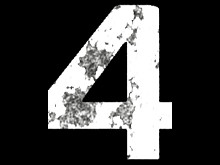The image displays a small, landscape-oriented rectangle with a black background. Dominating the center is a large, white number 4, which is blocky and stylized with a triangular shape rather than simple line strokes. This number appears to have a concrete-like texture, disrupted by dark, etching-like black patches or stains, resembling broken bricks or water spills. These patches are primarily on the left-hand side of the number. The number 4 stretches the full height of the image, making it highly prominent against the dark backdrop.